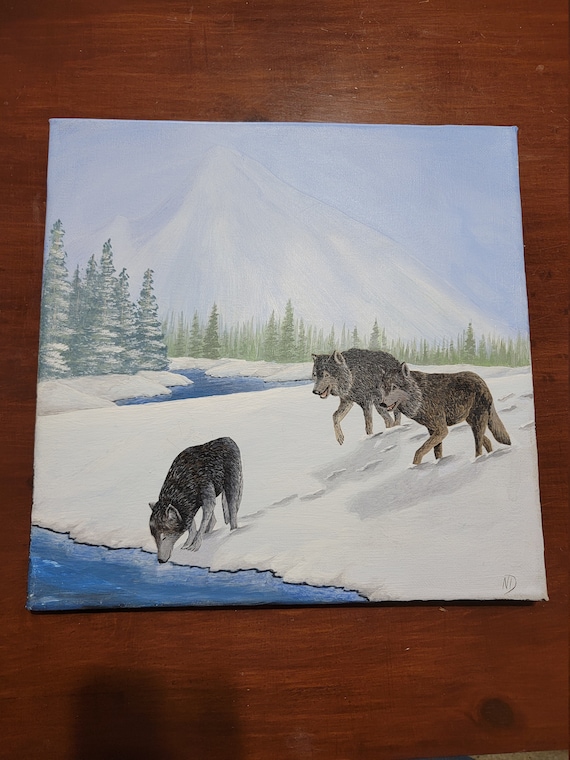The image depicts a detailed and serene winterscape painting resting on a wooden countertop. The central focus is on three wolves making their way through a snowy landscape. In the foreground, a gray wolf drinks from a winding stream, while two brown wolves follow behind, leaving faint paw prints in the snow. The background reveals a blend of green and snow-capped pine trees leading up to a grand, snow-covered mountain under a light blue sky. Notably, there are variations in the tree coverings, with some trees heavily laden with snow, especially to the left side of the painting. The stream appears to wrap around, hinting at multiple water bodies or a meandering brook. An artist's signature is subtly placed in the bottom right corner of the painting, providing a final touch to this tranquil winter scene.